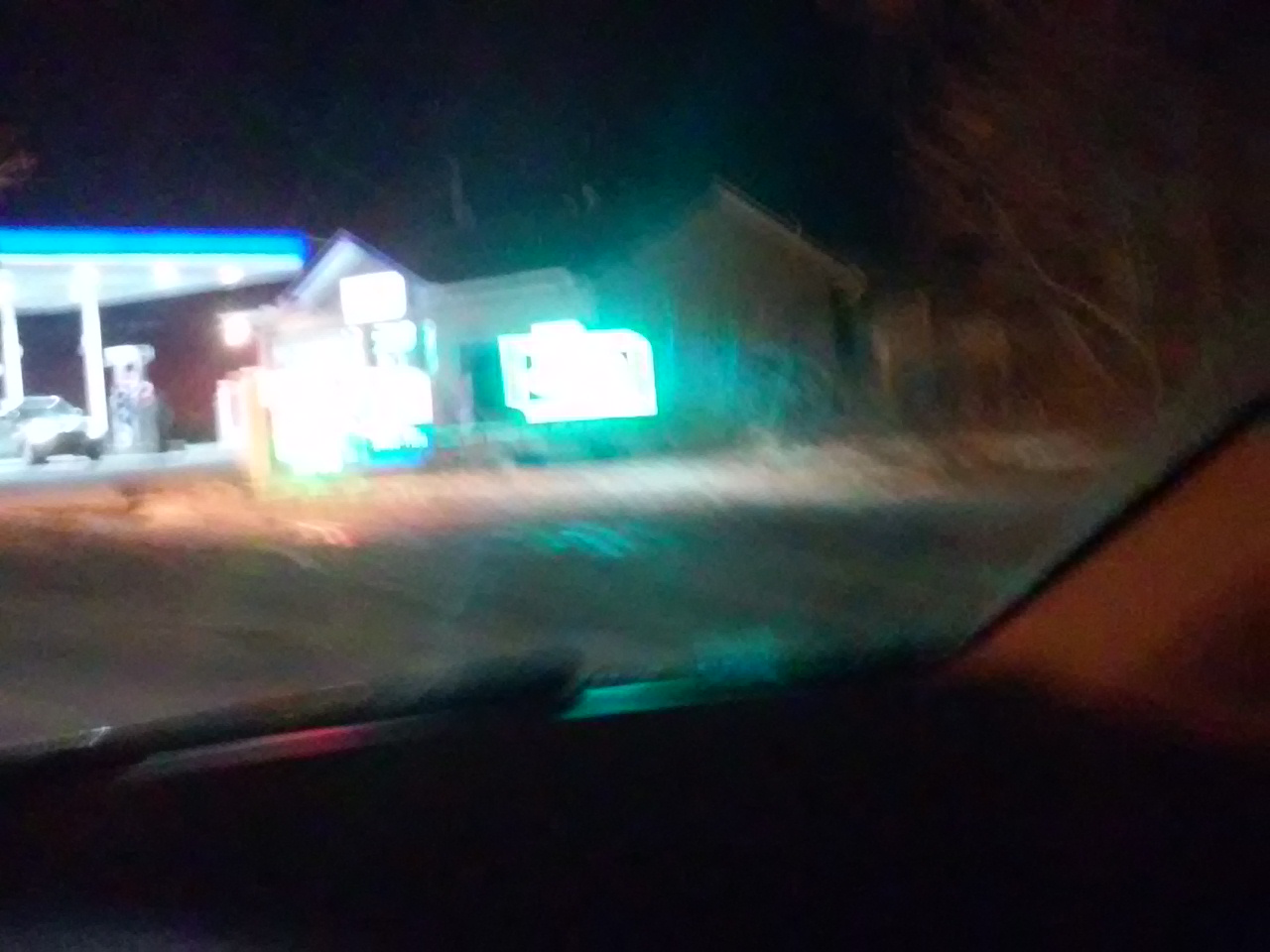Captured from inside a vehicle on a quiet night, this image provides a glimpse of a modest gas station bathed in a gentle glow. The scene is set at a smaller, less prominent establishment rather than a major retail chain. The convenience store, slightly obscure and blurry in the dim light, has a few illuminated signs, though their details are indistinguishable. The shelter of the gas station is visible, with one prominently featured car beside a pump, while another pump peeks into the frame. No other cars are present at the pumps, emphasizing the tranquility of the late hour. A lone tree is faintly visible off to the side, adding a touch of nature to the otherwise subdued urban landscape.